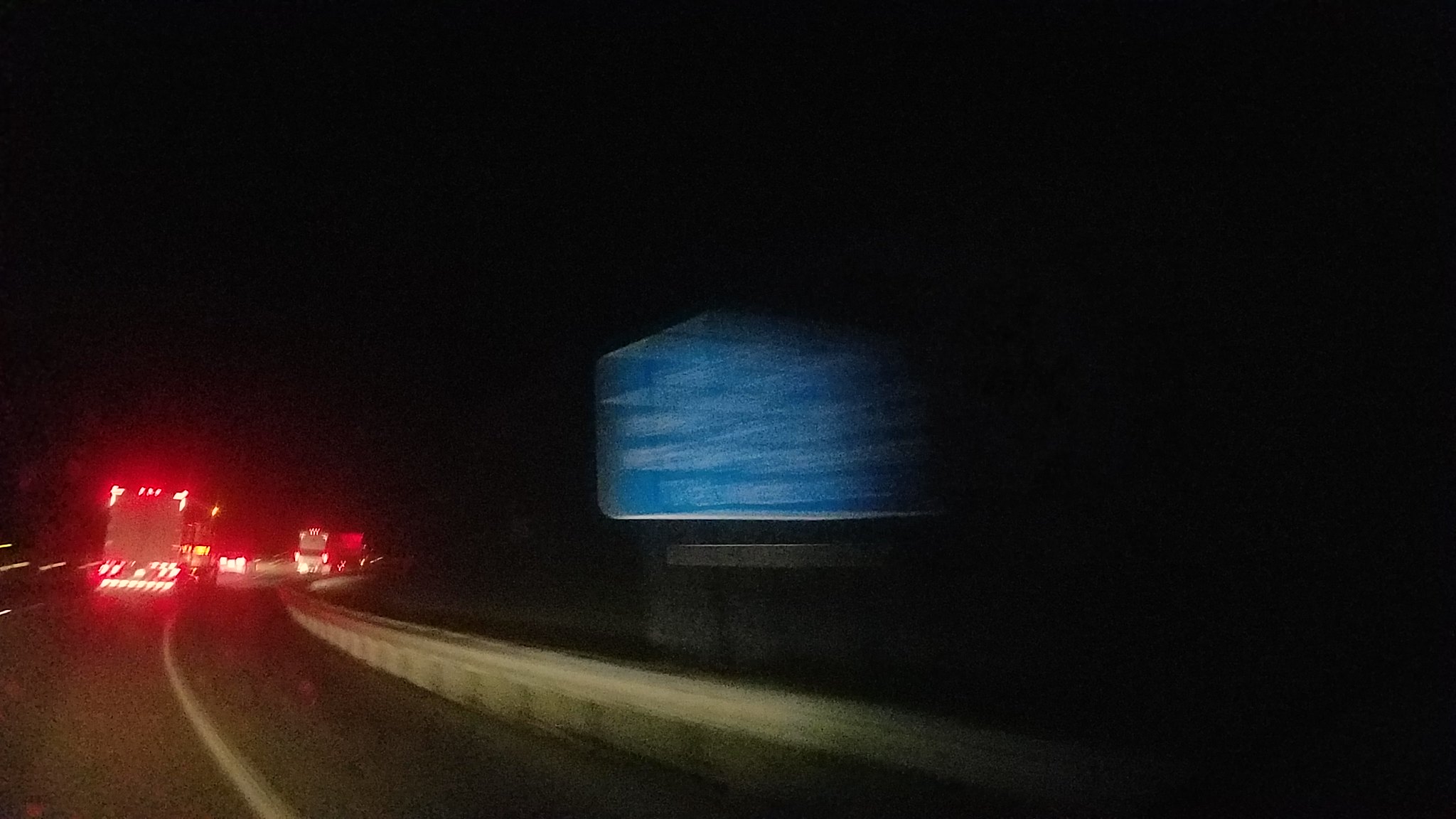A nighttime photograph captured from a moving vehicle, possibly by either the driver or the passenger. The image showcases an asphalt road marked by a white line running along the side. A guardrail lines the road, reflecting the light from the vehicle. On the right side, there's a blue sign with a white border and indiscernible white text, blurred due to motion. In the distance, several vehicles can be seen, all with illuminated red brake lights, suggesting a momentary halt in traffic. Among them are two large trucks and what appears to be a smaller sedan. The scene conveys a sense of movement and the quiet intensity of night driving.